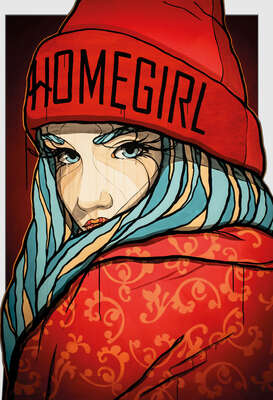The image depicts a cartoonish figure of a girl who is the central focus. She has striking hair that features blue, white, and beige or blonde stripes, matching her equally vibrant blue and white striped eyebrows. Her bright blue eyes, accentuated by very long, spider-leg-like eyelashes, give her a piercing gaze as she glances over her left shoulder. Her face is peach-toned with rosy red lips. She wears a red hat with the word "Homegirl" emblazoned on the front and a red jacket adorned with ornate orange and yellow floral prints. The background is a gradient of dark reddish-black, and there are a few thin artistic lines scattered across the image, adding to its detailed composition. A white border frames the upper portion of the picture, further highlighting the character.